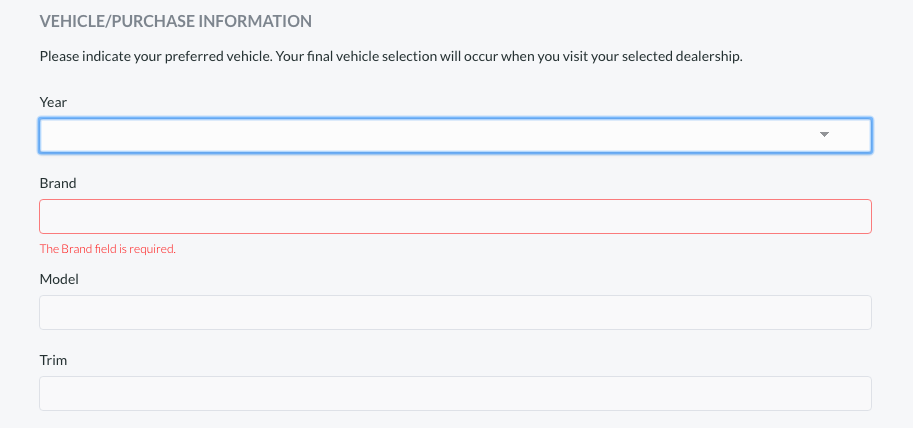The image features a light gray background with a user interface form for vehicle purchase information. At the top left, "VEHICLE / PURCHASE INFORMATION" is prominently displayed in dark charcoal font and capital letters. Directly underneath, an instruction reads, "Please indicate your preferred vehicle. Your final vehicle selection will occur when you visit your selected dealership."

Below the instruction, the form presents several dropdown menus and text fields:
1. **Year**: This field is outlined with a blue border and includes a downward-pointing arrow on the right end, indicating a dropdown menu.
2. **Brand**: This field is outlined in red with a note in red text beneath it stating, "The Brand field is required." The "T" in "The" and the "B" in "Brand" are capitalized.

Following the brand field, there are additional input fields for the vehicle's details:
- **Model**: An open space is provided for entering the vehicle's model.
- **Trim**: Another open space is presented to input the vehicle's trim level.

Each label for the fields—"Year," "Brand," "Model," and "Trim"—begins with a capital letter. The overall design is clean and structured, guiding the user through the process of specifying their preferred vehicle details efficiently.